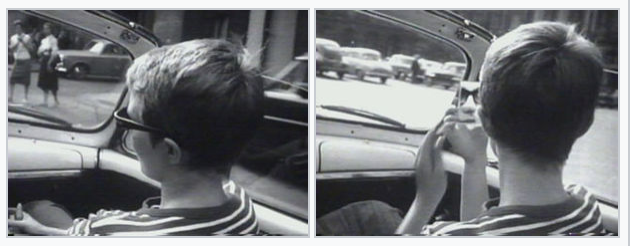This black-and-white image is a large rectangular photo, split into two side-by-side square photographs with a thin white border between them. Both photos capture the same boy seated in the passenger seat of a vintage convertible car, emphasizing the historical feel of the 1950s or 60s. 

In the left image, the boy sits with his hands crossed on his lap, wearing dark sunglasses and a horizontally striped shirt. Two women can be seen outside the vehicle, dressed in white shirts and black skirts, standing near another vintage car that hints at the era. 

The right image offers a slightly different angle, showing the boy holding up a mirror in which his sunglasses and a part of his nose are reflected. His head is turned to the right, giving a clearer view of the row of vehicles in front of him through the car’s open top. This detailed composition portrays a nostalgic scene, possibly capturing a candid moment from a bygone era.